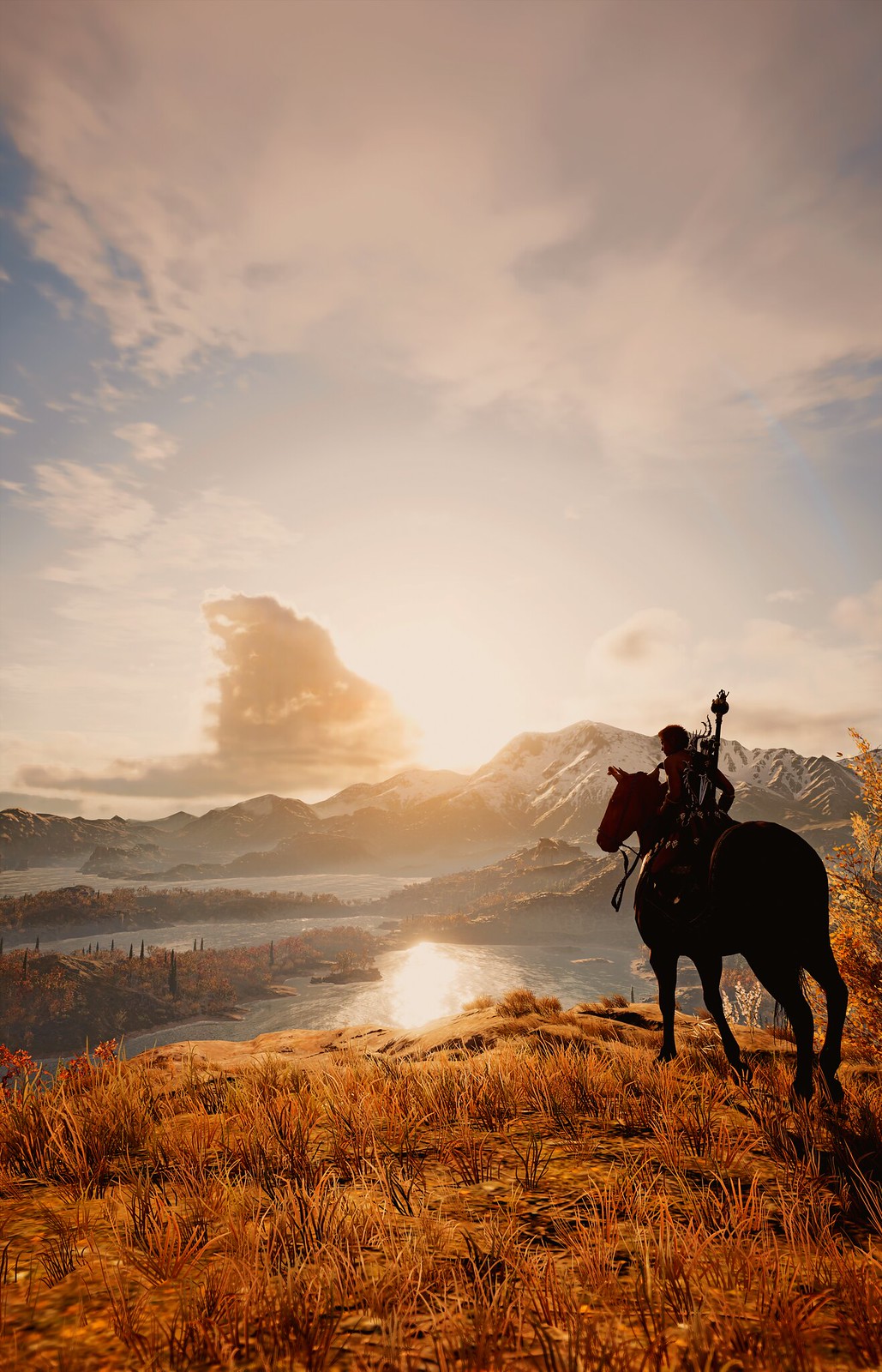In this evocative photograph, a shirtless individual sits astride a horse positioned on the edge of a cliff. Draped over their shoulder is a cloth, and they appear to be carrying weapons. The horse stands on a carpet of yellow-brown grass that stretches to the brink of the precipice, overlooking a serene body of water glistening with reflected sunlight. Majestic, snow-capped mountains rise in the distance, framed by a clear blue sky dotted with wispy clouds. The Sun peeks out from behind the mountainous backdrop, casting a warm, golden hue over the scene. Below the cliff, patches of orange-tinged grass and glimpses of trees can be seen, enhancing the image's rich, natural tapestry.